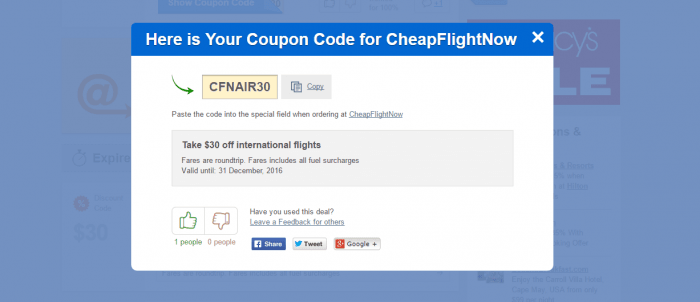The image depicts a computer screen with a predominant blue rectangle as the background. Through the semi-transparent blue overlay, a red area suggesting a Macy's Day sale is partially visible. However, a white rectangular pop-up obscures part of this backdrop. At the top of the pop-up, a thin blue strip features the message "Here is your coupon code for cheap flight now" in white text, accompanied by an 'X' icon on the far right to close the window.

Below this heading, a yellow box prominently displays the coupon code "CFNAIR30," highlighted by a green arrow curving downward to point at it. Further down the pop-up, text informs viewers of a "$30 discount on international flights," explaining that the fares are for round trips and include all fuel surcharges. The offer is noted to be valid until December 31, 2016. At the bottom of the pop-up, social feedback is shown with one person giving a thumbs up and none giving a thumbs down.